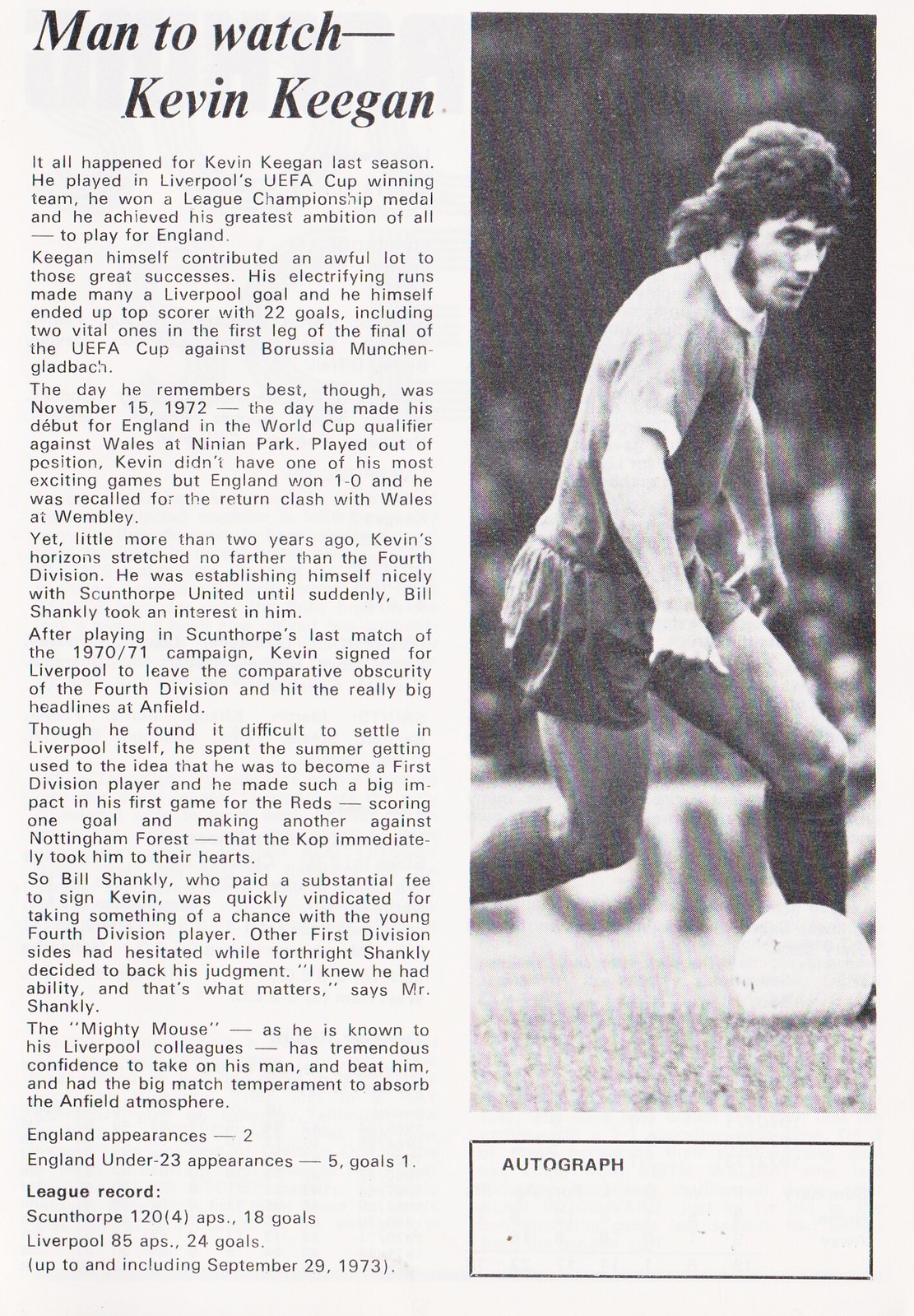The black-and-white newspaper article, titled "Man to Watch: Kevin Keegan," features an in-depth profile of the soccer player Kevin Keegan. The article is divided into two sections: the left-hand side containing detailed text about Keegan's career and achievements, and the right-hand side showcasing a full-length photograph of him. The image presents Keegan dressed in mid-thigh shorts, a dark-colored soccer jersey, and dark-colored socks, with the soccer ball positioned under the instep of his left foot as he appears ready to kick with his right leg bent behind him. He sports a mullet hairstyle and a chin-strap beard. Below the picture, the word "AUTOGRAPH" is prominently printed in capital letters.

The article covers Keegan's rapid rise in football, highlighting his breakthrough season with Liverpool during which he played a crucial role in winning the UEFA Cup and the league championship. It recounts his debut for England in a World Cup qualifier against Wales and his transition from the 4th division to becoming a beloved figure at Liverpool under manager Bill Shankly. Keegan's energetic playing style and scoring prowess earned him the nickname "Mighty Mouse" from his teammates. The piece concludes with a summary of his career statistics, including appearances and goals for both club and country up to September 29, 1973.